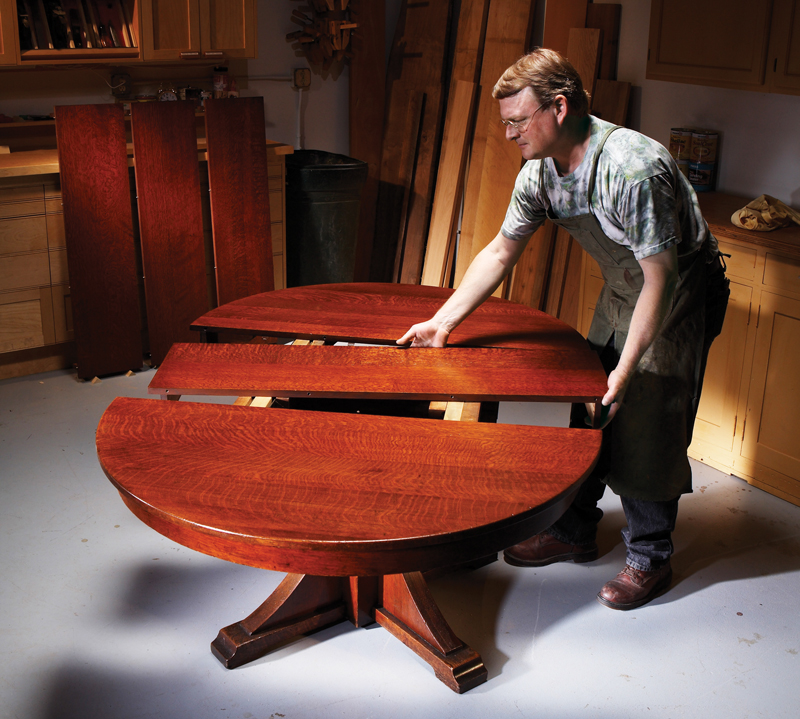The image captures a detailed scene inside a woodworker's workshop or garage, where a man is in the process of expanding a circular dining table. The table, crafted from polished, tan cherry wood, is currently opened up as the man carefully places an extender in its middle section, transforming the table from a circular to an oval shape to accommodate more seating. He is wearing a dark green full-length apron over a tie-dye styled blue and green t-shirt, paired with baggy blue jeans and brown work boots. The man has brown hair combed to the side and wire-rimmed glasses, emphasizing his focused demeanor. In the background, various wooden planks of different lengths and widths are neatly stacked, alongside three other table leaf extenders that match the one he is positioning. The workspace also features cabinets in a lighter brown shade and some more wood stacked in the back corner. The floor is gray, further highlighting the workshop’s practical, industrial atmosphere.